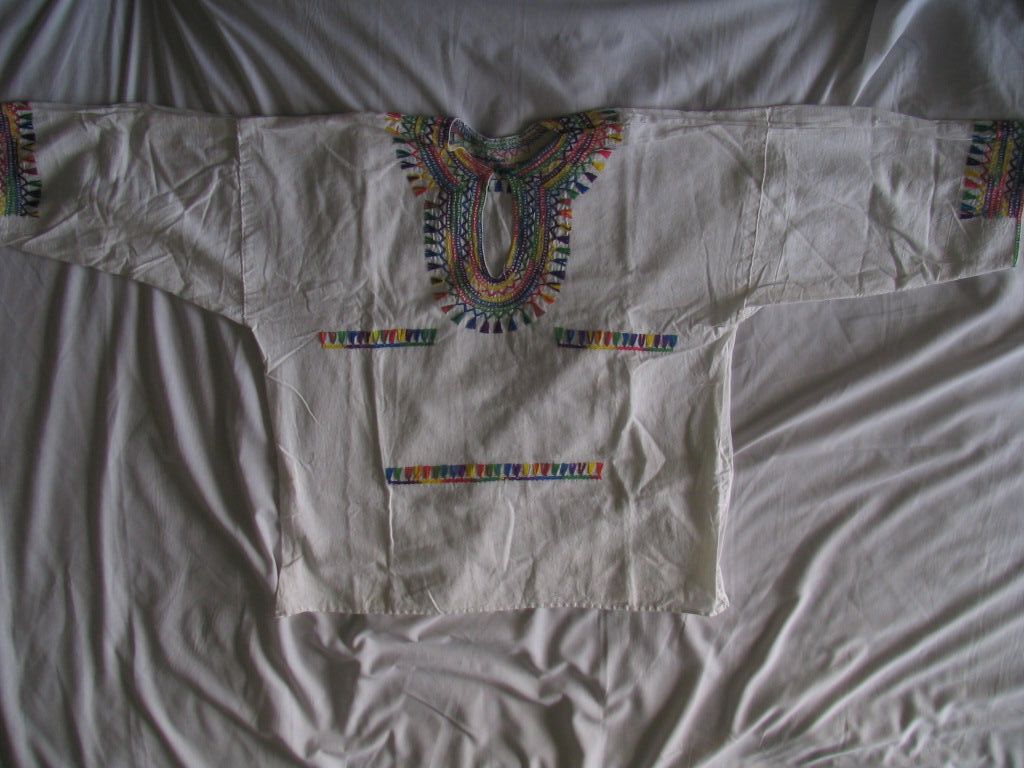The image displays a white, long-sleeved shirt adorned with intricate, hand-knitted rainbow-colored accents. These accents include horizontal stripes located on either side of the chest and a longer stripe centered below them, resembling a sort of smiley face. Additional colorful, embroidered designs featuring blues, reds, yellows, greens, and purples decorate the neck collar and sleeves. The shirt appears to be considerably wrinkled and is laid out on a similarly wrinkled white sheet. The photograph is relatively dark, suggesting it was taken in a shaded room. Both sleeves are fully extended, and the shirt is presented in a way that suggests careful arrangement on a fabric surface.